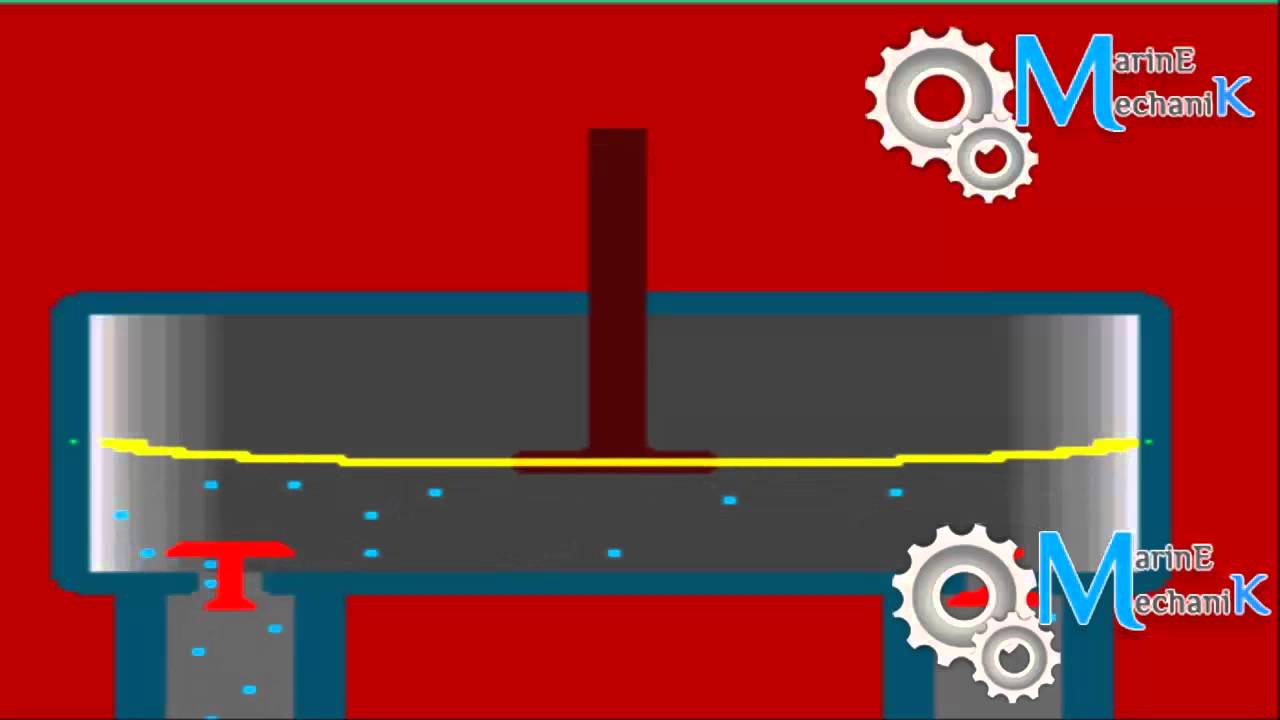The image displays a digital diagram set against a vivid red background, featuring two identical logos labeled "Marine Mechanic," with "Mechanic" notably ending in a bright blue 'K'. Both logos, each adorned with a large light blue 'M', are positioned at the top right and bottom right corners, partially overlaying other elements of the diagram.

Central to the image is a complex structure resembling a sink, characterized by a long gray horizontal rectangle with two shorter, horizontal rectangles or pipes extending downward. A prominent yellow horizontal line traverses the middle of the sink-like structure, stopping a collection of small blue dots from rising above it. Above the yellow line is a thinner brown rectangle, possibly a plug, further preventing the blue dots from moving upward.

Below the yellow line, the blue dots are concentrated in the lower portion of the structure and seem to be channeling downwards through the two pipes. The pipes feature red T-shaped plugs at their ends, which adds to the visual impression of controlling the movement or flow of the blue dots.

The blend of colors, including magenta, crimson red, blue, and gray, enhances the intricate design and functionality depicted in the diagram. The repeating logos and vivid background draw attention to the detailed technical illustration, suggesting its relevance to marine mechanics.